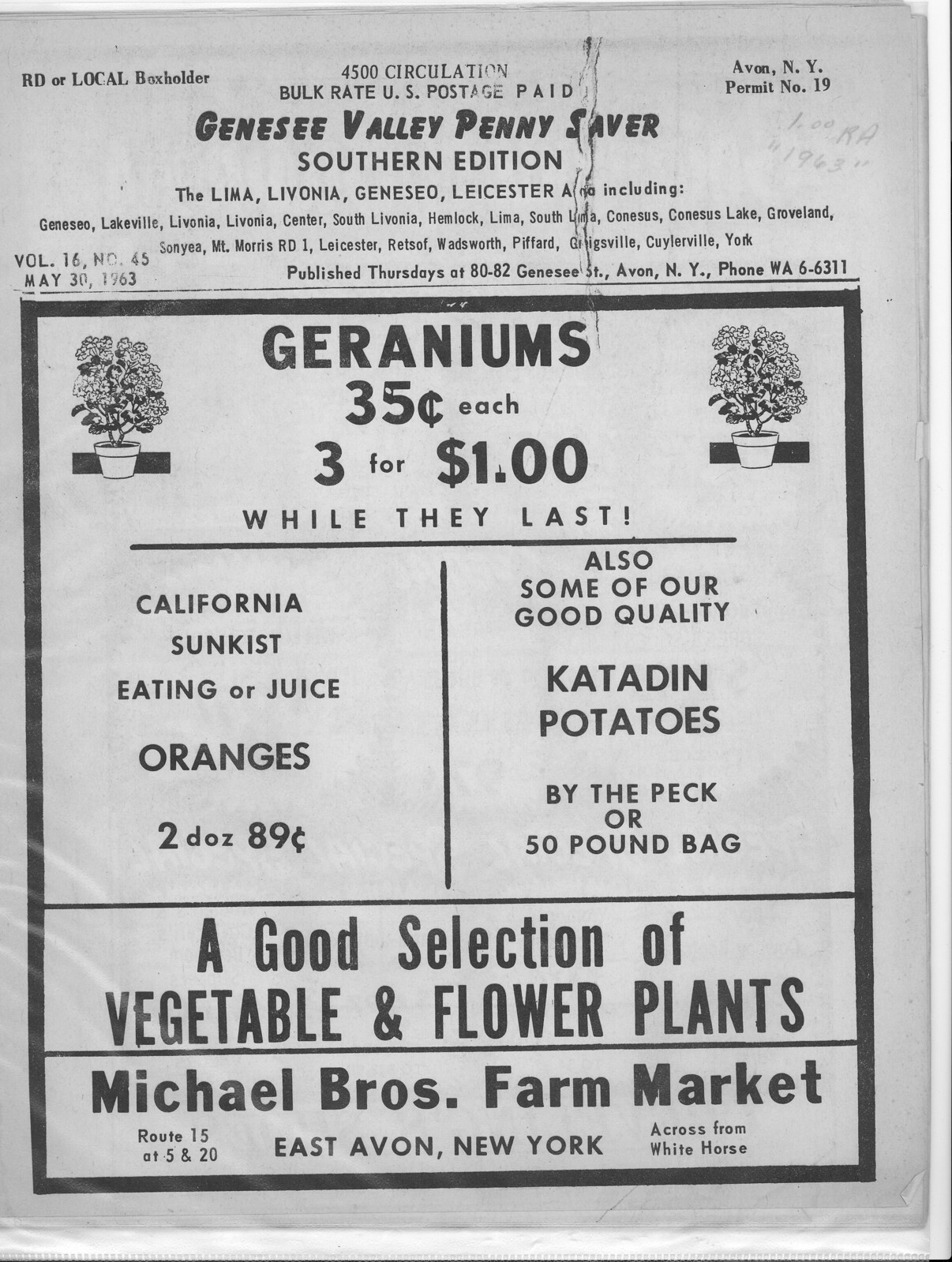This is the front cover of a vintage Genesee Valley Penny Saver, Southern Edition, which serves the Lima, Livonia, Geneseo, and Leicester areas. The background is white with a black frame along the upper left and right sides. At the top, text in capital letters reads "RD or Local Box Holder." Below that, in tiny font, it mentions "4500 Circulation, Bulk Rate U.S. Postage Paid," followed by "Avon, New York, Permit Number 19" to the right.

Prominently displayed in larger, bold letters is "Genesee Valley Penny Saver, Southern Edition." Below this, it states, "Published Thursdays" along with "80 to 82 Genesee Street, Avon, New York" and includes a phone number. The date "May 30th, 1963" is also noted along with a volume number.

Central to the design is an advertisement featuring illustrations of geraniums with the text, "Geraniums, 35 cents each or three for $1 while they last." To the side of this, there's a promotion for California Sunkist eating or juice oranges, priced at "2 for 89 cents." Additionally, it highlights "Good quality Katahdin potatoes by the peck or 50-pound bag," as well as "A good selection of vegetable and flower plants" available at Michael Brothers Farm Market. The market's location is specified as being on "Route 15 at 5 and 20 in East Avon, New York, across from White Horse."